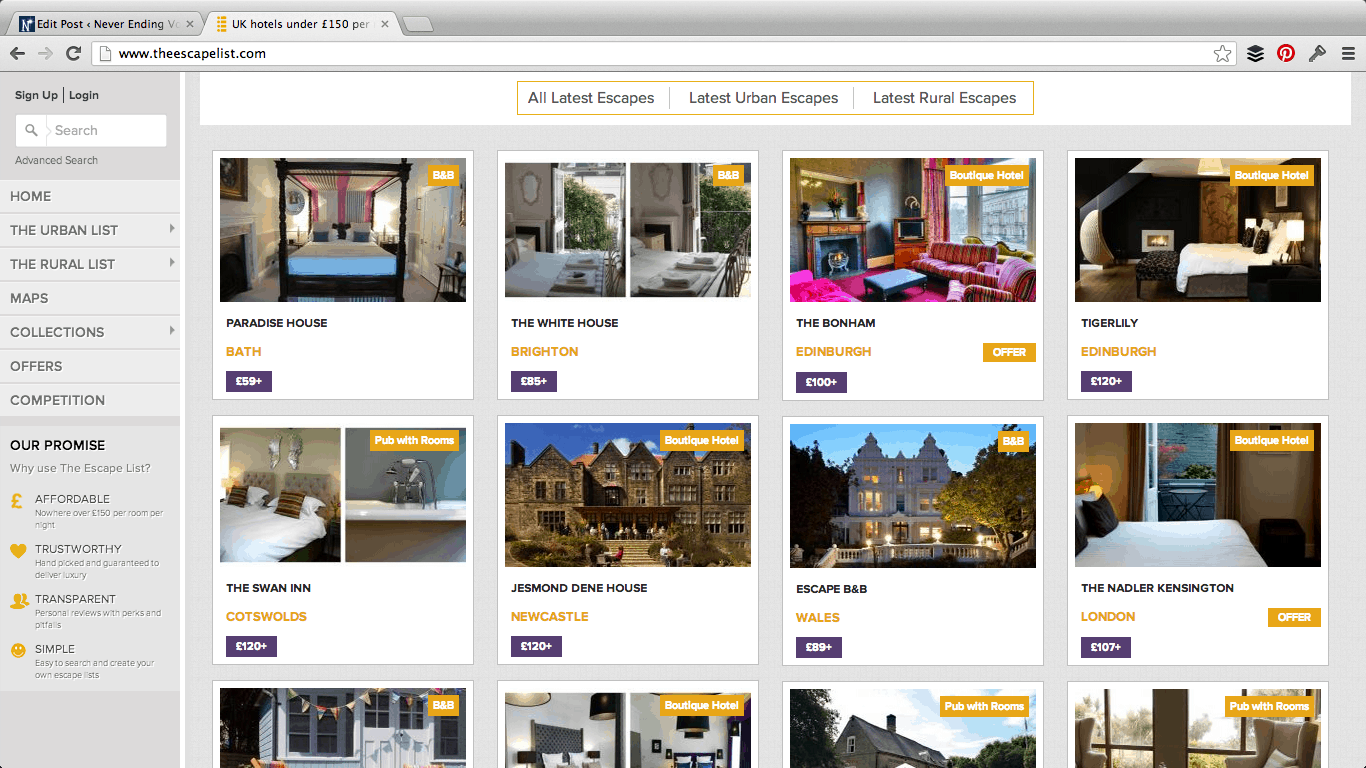The image displays two tabs open in a browser. The tab on the left reads "Edit Post - Never Ending," while the active tab shows a search result titled "UK Hotel Under 150 Pounds." The content within this tab is organized into a grid layout featuring 12 hotel options, displayed in three rows of four images each. However, the bottom row is partially cropped, only revealing the top halves of those images.

The descriptions of the hotels, from the top left to the bottom right, are as follows:
1. Paradise House, Bath - £59
2. The White House, Brighton - £85
3. The Bonham, Edinburgh - £100
4. Tiger Lily, Edinburgh - £120
5. The Swan Inn, Cotswolds - £120
6. Jetman Dean House, Newcastle - £120
7. Escape B&B, Wales - £89
8. The Nadler Kensington, London - £107

Additionally, there is a navigation list on the left side of the screen with the following options: Home, The Urban List, The Rural List, Maps, Collection, Offer, and Competition.